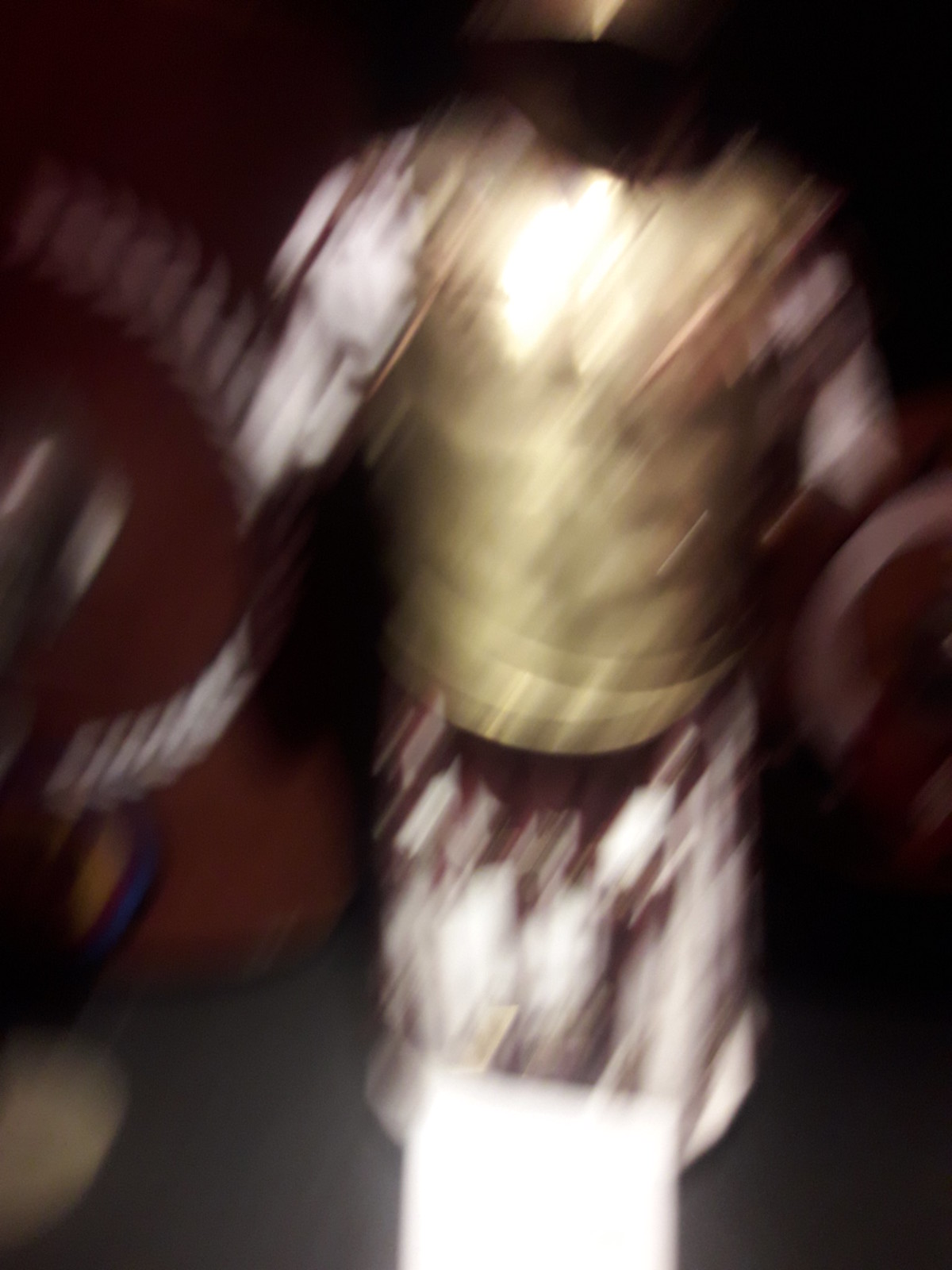The image depicts a statue of a knight adorned in full armor, though the picture is somewhat blurry. The knight is outfitted with a glistening gold helmet and a matching gold chest plate that spans from the shoulders down to the waist. The arms of the statue appear slightly out of focus but are clad in silver armor, as are the legs, creating a striking contrast between the two metals. The background of the image is completely black, enhancing the knight's imposing presence. A square white light or object is noticeable at the bottom center of the image. Additionally, there is a notable reflection on the upper chest of the breastplate, adding a touch of realism and depth to the statue’s depiction.